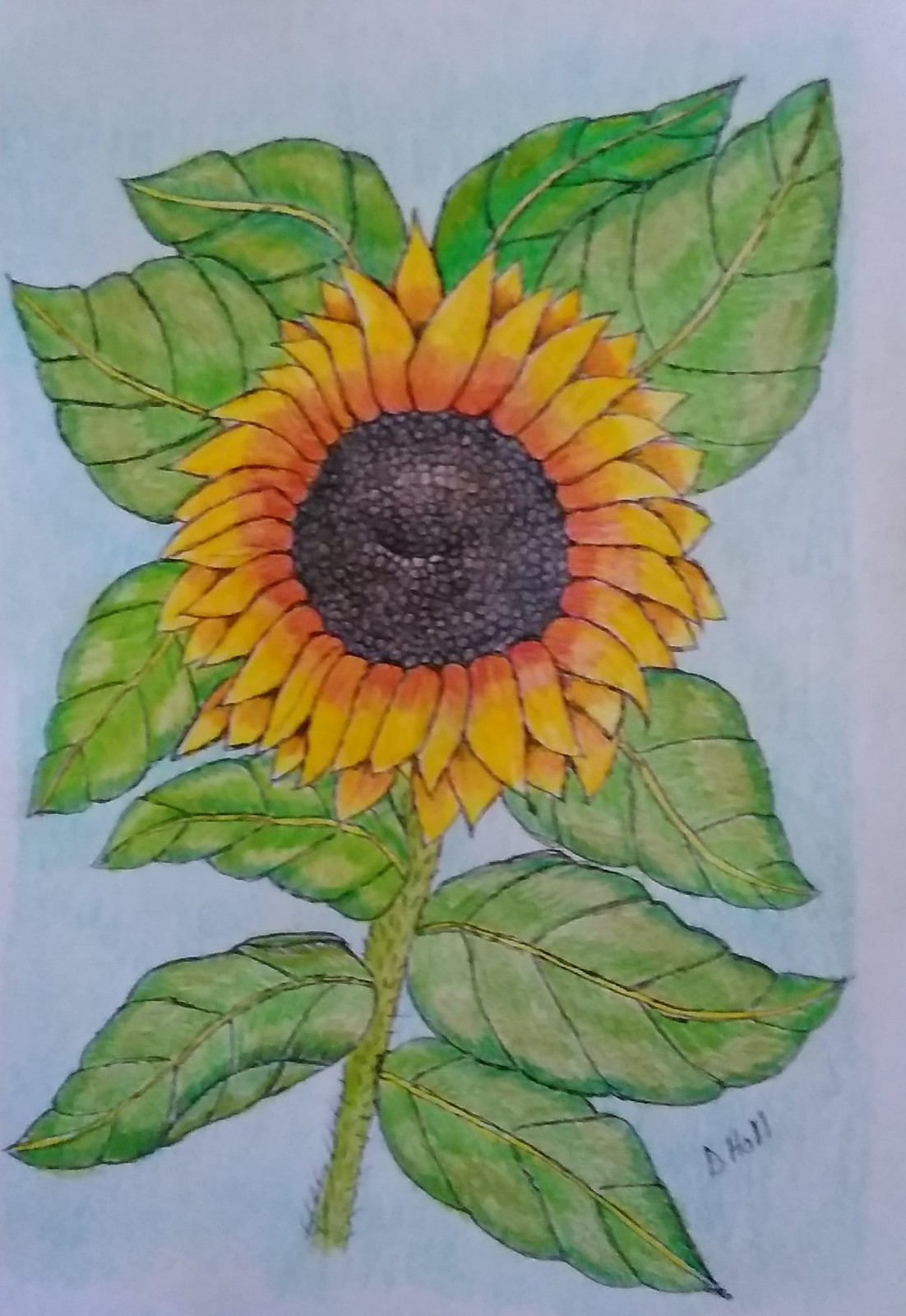This is a highly detailed colored pencil drawing of a vibrant sunflower, crafted meticulously on a pale blue-lavender piece of paper. The sunflower's stem, rendered in a delicate pale yellowish-green hue, exhibits small bristles, enhancing its realistic texture. Four pointed leaves extend symmetrically along the stem, each intricately detailed with a prominent center vein and smaller side veins that extend to the edges. The sunflower itself is a burst of color, with golden petals transitioning to a warm orange near the flower's core, culminating in a richly textured dark brown center dotted with small nubs.

Above the sunflower, additional leaves echo the design and detailing of those below. The overall composition exudes a sense of natural beauty and artistic finesse. In the far right corner of the paper, the artist has signed their work with the initial and last name, "D. Hall," adding a personal touch to this exquisite botanical illustration.